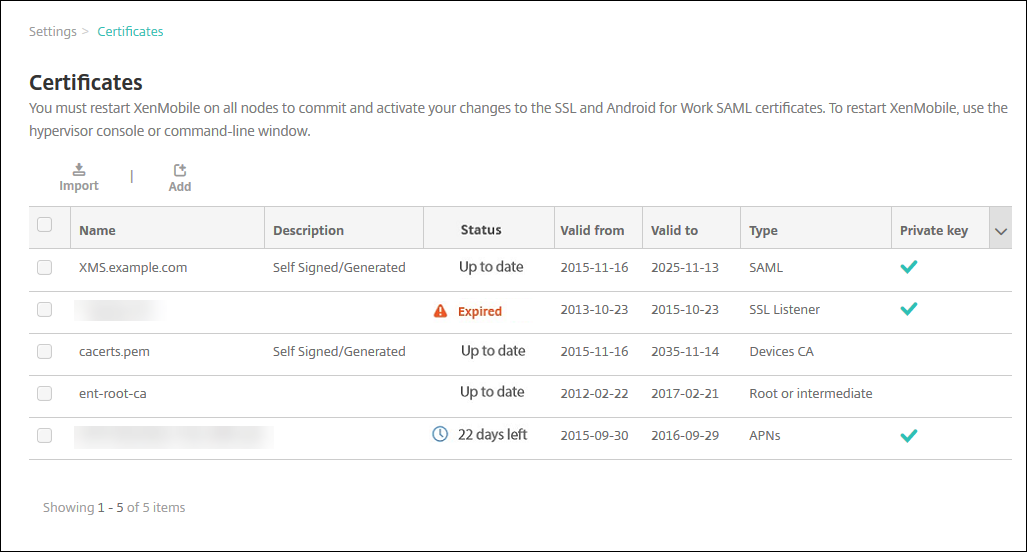This horizontal rectangular image presents a detailed display within a settings interface. The top section features a breadcrumb trail with "Settings" in light gray, followed by a greater-than sign, and "Certificates" in bright green, all set against a white background framed by a black border.

Below this, "Certificates" is prominently displayed in black bold font. Underneath, a message in regular bold gray font reads: "You must restart Zenmobile on all nodes to commit and activate your changes to the SAML and Android for Work SAML certificates. To restart Zenmobile, use the hypervisor console or command-line window."

Further down, two icons labeled "Import" and "Add" appear, followed by a neatly divided chart. The leftmost column of the chart contains empty squares. The header row, in bolded gray font, lists the categories: "Name", "Description", "Status", "Valid From", "Valid To", "Type", and "Private Key".

The first row under "Name" displays "XMS.example.com". The "Description" column shows "Self-signed\generated". The "Status" is marked "Up to Date" with specific validity dates under "Valid From" and "Valid To". In the "Type" column, it reads "SAML" with a check mark under "Private Key".

The second row is partially whited out. Its "Status" indicates "Expired" in orange with an orange triangle containing a white exclamation point. The "Type" is listed as "SSL Listener" with a check mark.

The third row shows "CACERT.PEM" in the "Name" column, "Self-signed\generated" in "Description", and "Up to Date" under "Status". It is labeled "Devices C-A" in the "Type" column, but lacks a check mark under "Private Key".

The fourth row is "ENT.root.CA", marked as "Up to Date" with specified dates and categorized as "Root or Immediate" in "Type", also without a check mark.

The final row, partially whited out, displays "22 days left" under "Status" with a blue clock icon beside it. The "Type" is "APNs," and there is a green check mark under "Private Key".

This image provides a comprehensive look at the certificate management section within a settings interface, detailing each certificate's status, type, and validity.